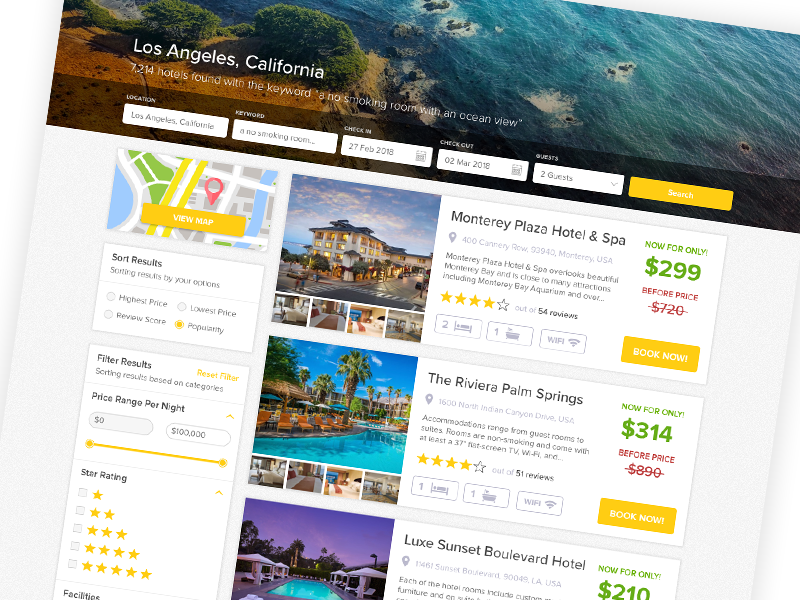The image showcases a travel-themed website interface, slightly angled to the right. The top banner features an aerial photograph of a waterfront, capturing a serene body of water adjacent to a brownish shoreline, fringed with patches of grass and bushes. Overlaying the image, text reads "Los Angeles, California" and announces that "7,214 hotels found." Below the banner, the section displays a comprehensive search tool. Notably, it includes a message indicating "No smoking rooms with an ocean view," followed by a search bar complete with five pull-down options. The first two options appear to be input fields. In the lower section of the page, initial search results of the hotels are visible, detailing the accommodations available in Los Angeles.